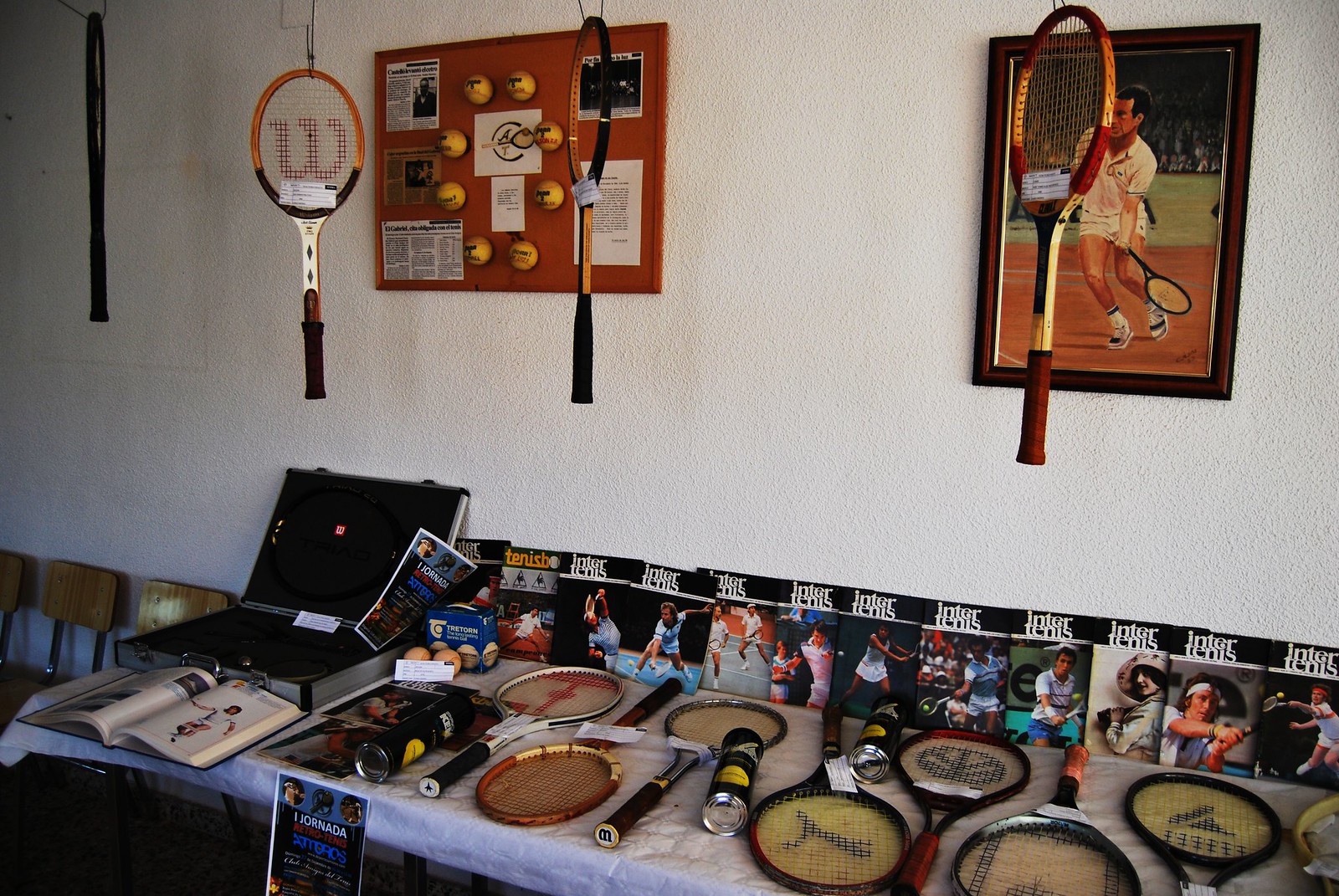The image depicts a detailed indoor display dedicated to tennis memorabilia. Dominating the scene is a long, rectangular table covered with a white plastic tablecloth, set against white textured walls. Scattered across the table are several vintage tennis rackets with black handles and varying colored strings—red, yellow, and white—and containers of yellow tennis balls. An open book and a small silver suitcase are prominently placed on the left side of the table.

On the wall above the table, numerous framed photographs and paintings of tennis players in action are displayed. A notable framed painting of what might be John McEnroe swinging at a tennis ball is evident. A cork bulletin board with a vivid orange backing is adorned with newspaper articles and encircled by tennis balls. 

Several tennis rackets are hung both on the wall and from the ceiling via hooks, creating a dynamic visual layer. In one corner, a meticulous arrangement of chairs is seen. The overall setup suggests this is a passionate collector's homage to the sport, featuring an assortment of tennis items that evoke a sense of nostalgia and celebration of tennis history.